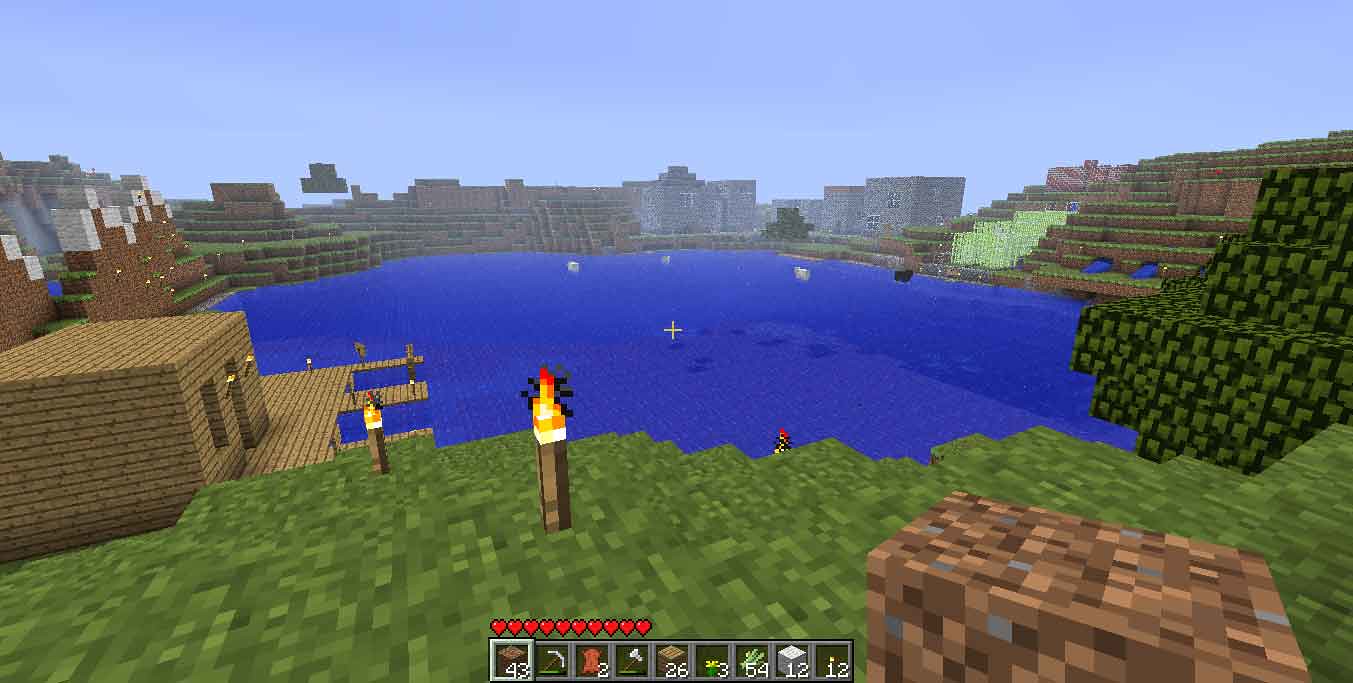This is a screenshot from Minecraft showcasing a serene, expansive lake marked by a central cursor crosshair. The foreground features lush green grass sloping gently towards the tranquil lake, where the vibrant blue water reflects the surrounding landscape. Dominating the scene is a large, intricately designed brown building constructed from various shades of brown blocks, enhancing its textured appearance.

Flanking this central structure, two prominent towers rise majestically, built from brown bricks and topped with flaming torches, adding a medieval flair to the hillside view. To the left, another structure adorned with torches exudes warmth, casting a gentle glow over the area.

Encircling the lake are multiple buildings and a series of tiered steps, each level edged with verdant grass, reminiscent of a grand amphitheater offering prime viewing spots of the lake's activity. In the water itself, indistinct shapes float—potentially boats, though their vague forms may also resemble cows. The overall scene is a harmonious blend of nature and human ingenuity, captured in the distinctive blocky style of Minecraft.